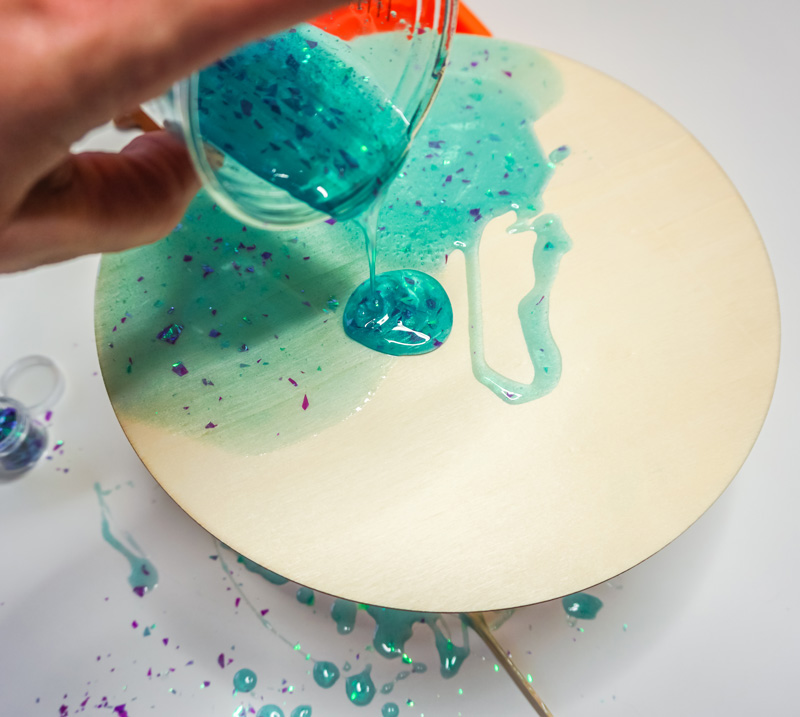A reddish-brown hand is captured in mid-motion, pouring a teal-colored, glittery liquid from a small glass beaker onto a slightly off-white wooden circular surface. The liquid splatters, forming droplets and streaks, some of which spill beyond the edges of the wooden surface, adding to the visual dynamic of the scene. This creative setup suggests an arts and crafts project, either for a child or an adult. The glittery liquid is speckled with darker blue particles, creating a mesmerizing effect. In the top middle part of the image, an indistinct orange object can be seen, hinting at other materials used in the craft. Additionally, a small blue glitter container is positioned towards the middle left of the scene. The activity unfolds on a white backdrop, highlighting the vibrancy of the teal liquid.